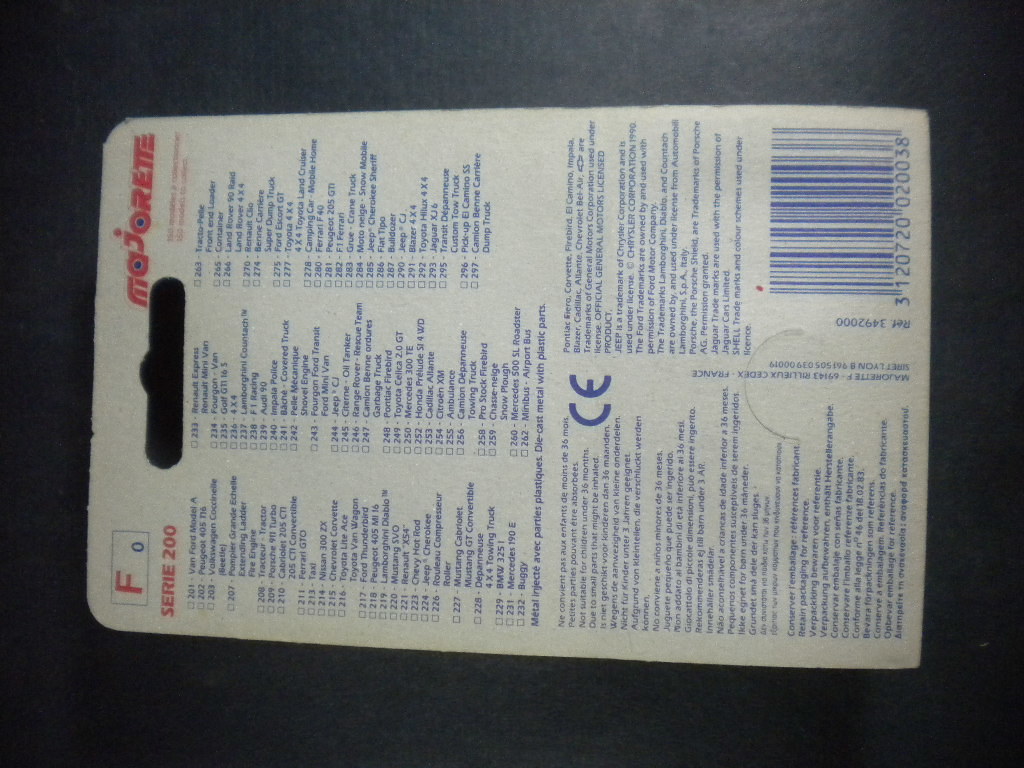The photograph depicts the back of a hang card for a product in a store, rotated counterclockwise by 90 degrees so that the top of the card is on the left and the bottom is on the right. At the top left of the hang card, there is a prominent red letter "F" with "Siri 200" written beneath it in red. To the right, in red letters, it says "MAJORETTE," and nestled between these two red-lettered sections is a punched-out area designed for hanging the card on a pegboard display.

The background of the hang card is white with numerous paragraphs of black text on its right-hand side. When properly oriented, the top left corner features a black-on-white UPC code. The card also contains blue print detailing various types of cars, including names like Van, Ford, Model A, Peugeot, Volkswagen, Porsche, Ferrari, Nissan, Chevrolet, and Toyota, among others. Centrally located, there's a CE logo, and the hang card's material suggests it might be closed and standing against a black surface, likely a table or shelf. The overall appearance indicates that the hang card serves as an informative guide, potentially for car models or related parts, complete with an arrangement for easy display.